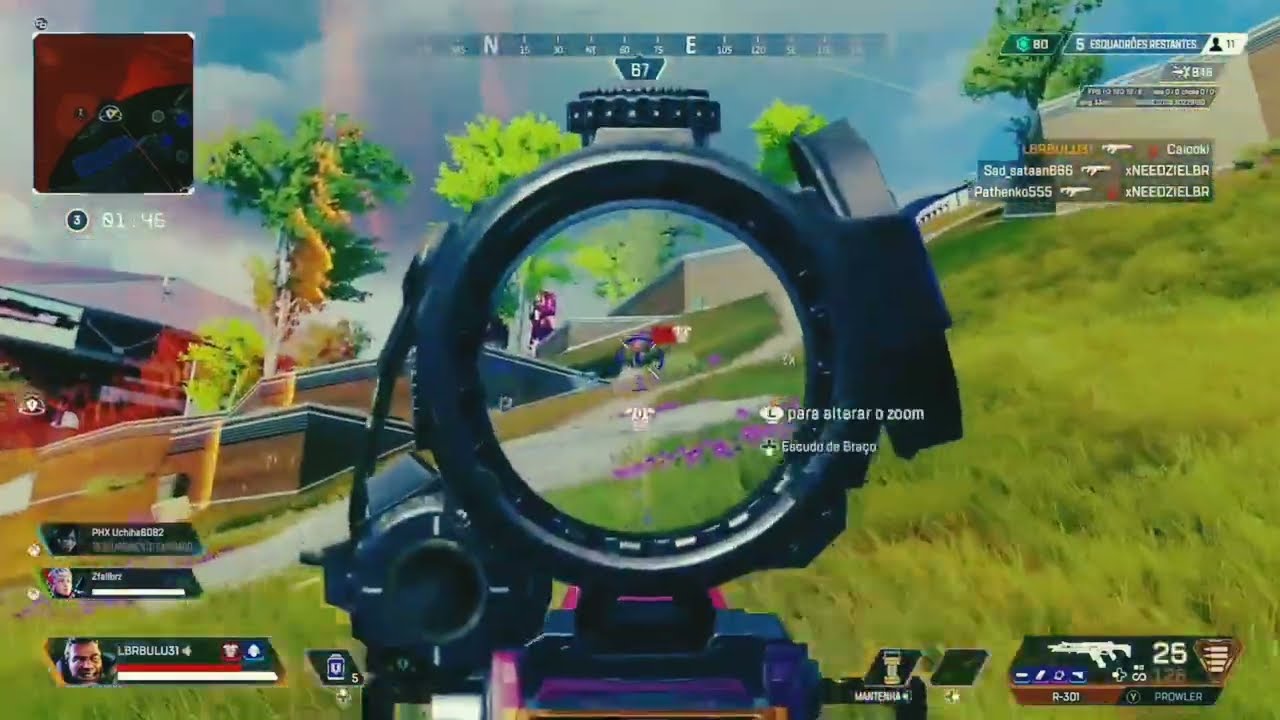The image is a detailed screenshot from a first-person shooter video game, depicting a player's perspective as if they are looking through a rifle scope at a distant target. The landscape features a grassy hill area with some trees, a concrete structure, and a white building to the right. The foreground includes the metal parts of the scope and a portion of the weapon, with the game interface displaying various informational elements. 

In the top left, there is a small square map with red and black colors, and beneath it a timer reading 1:45. At the top center, a compass indicating directions, specifically north and east, is visible. The sky in the background is blue, contributing to the vivid colors present throughout the scene. 

In the bottom right corner, there is a readout displaying the number 25 accompanied by a small image of a rifle labeled R-301 Prowler. The bottom left corner shows three avatars or player icons with faces, two of which have white lines beneath them. Additionally, a small image of a man is present with red and white lines next to him.

The top right corner contains text in another language with an icon of a person and the number 11. The overall scene is busy with various overlays and in-game elements that provide a rich and immersive gaming experience. A grassy patch is also visible in the foreground right, contributing to the natural aspect of the setting.